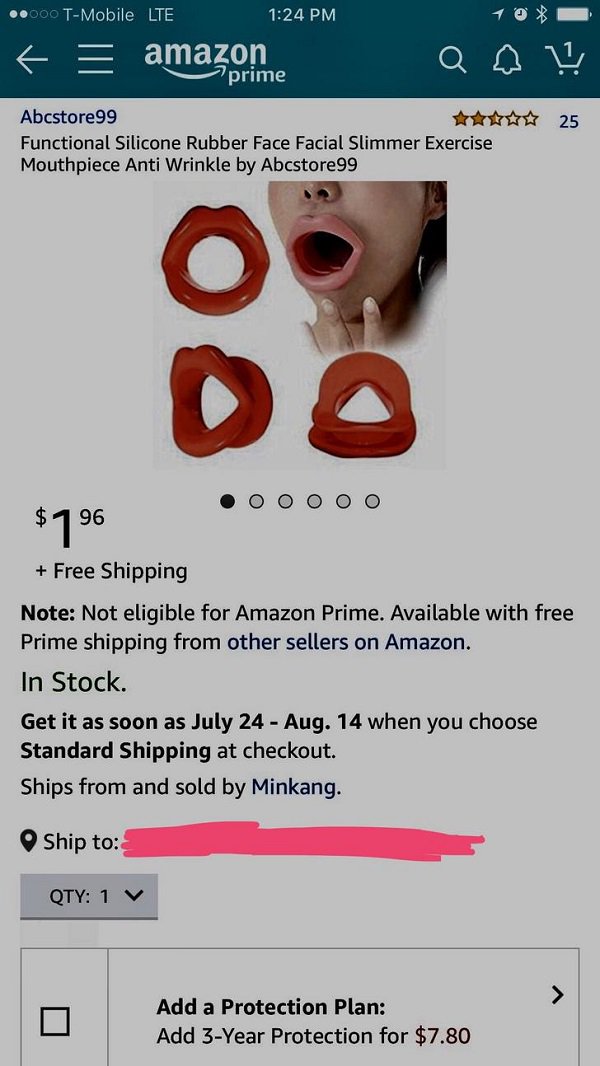Screenshot of Amazon Prime App Displaying Facial Slimmer Product

The image showcases a screenshot taken from an Amazon Prime app on a smartphone. At the very top, the status bar displays "T-Mobile LTE" with two out of five signal dots, the time "1:24 PM" at the center, and icons for an arrow, alarm clock, Bluetooth, and a fully charged battery on the right. Directly below, the navigation bar includes a left arrow, three horizontal lines, the Amazon Prime logo, a magnifying glass, a bell, and a shopping cart icon with a notification indicating one item.

The main content reveals a product listing from the ABC Store 99. The item displayed has garnered an average rating of 2.5 stars based on 25 reviews. The product is described as a "Functional Silicone Rubber Face Slimmer Mouthpiece Anti-Wrinkle", targeted at facial exercise and wrinkle reduction. Below the description, an image showcases three different silicone mouthpieces alongside a person demonstrating the product in use with one piece in their mouth.

The price is listed as $1.96 with the benefit of free shipping. A crucial note highlights that the item is not eligible for Amazon Prime directly but is available with free Prime shipping from other sellers on Amazon. Additional details indicate that the product is in stock and offers estimated delivery between July 24th and August 14th with standard shipping. The product is sold and shipped by MinKang, with the listing mentioning "quantity: one".